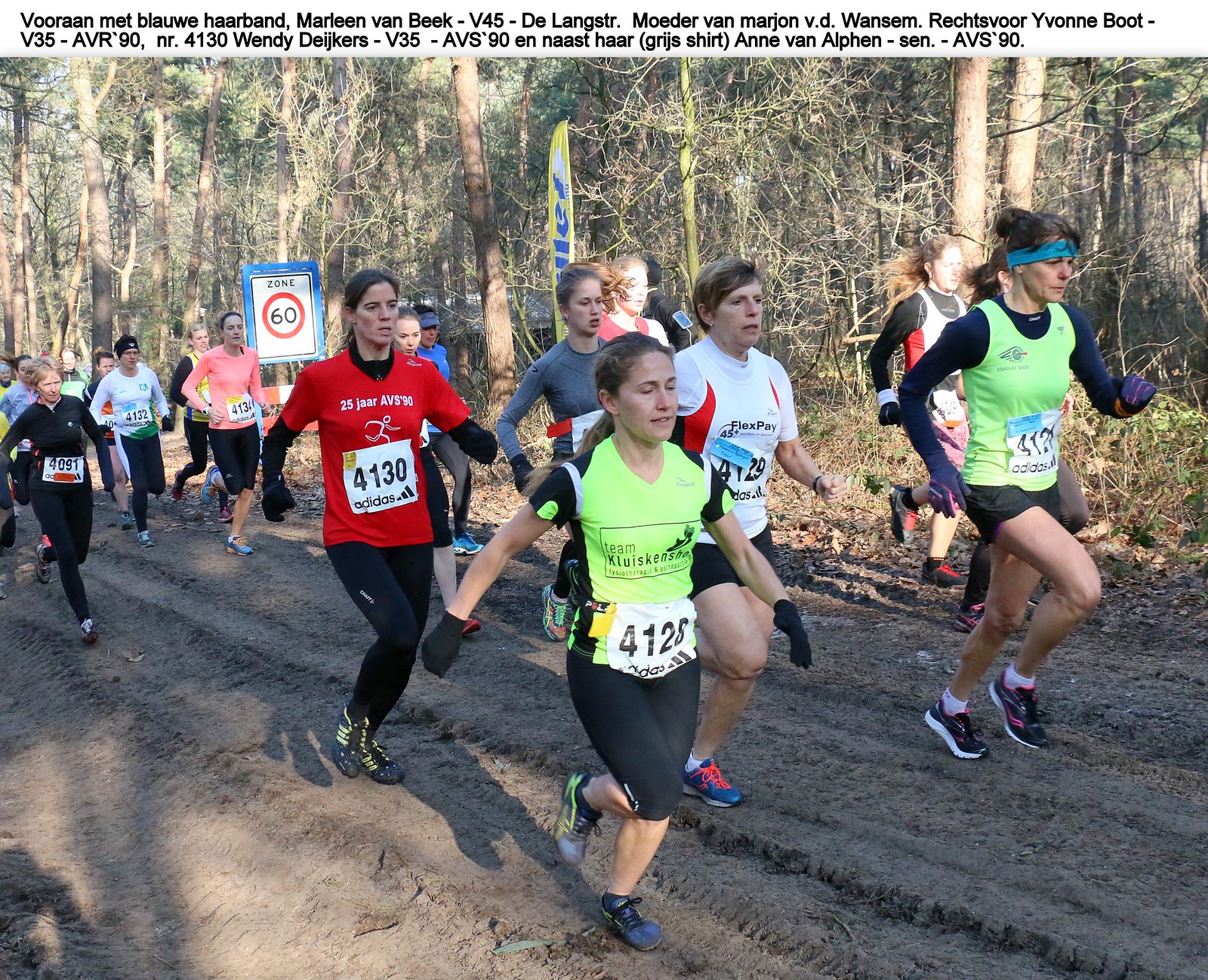This color photograph captures a group of approximately 16 to 18 women running a marathon on a muddy, tire-tracked path through a woodland setting with bare, leafless trees in the background. The runners are dressed in a variety of neon colors, spandex, and tight athletic wear suitable for cold weather, including short and long-sleeved shirts, gloves, headbands, and running shoes. Each woman has a numbered racing tag affixed to the front of their shirt, which also displays what appears to be the Adidas logo. The two leading women are distinguishable by their pale green shirts, with one wearing black shorts and the other in knee-length black pants, both also donning black gloves. Other runners are clad in colors such as red, white, pink, gray, and blue. Above the image, there is text in a foreign language, suggesting that the marathon is taking place in a country outside the United States, possibly in Scandinavia. The foreign text includes names and shirt numbers of the participants, hinting at runner statistics and race information.